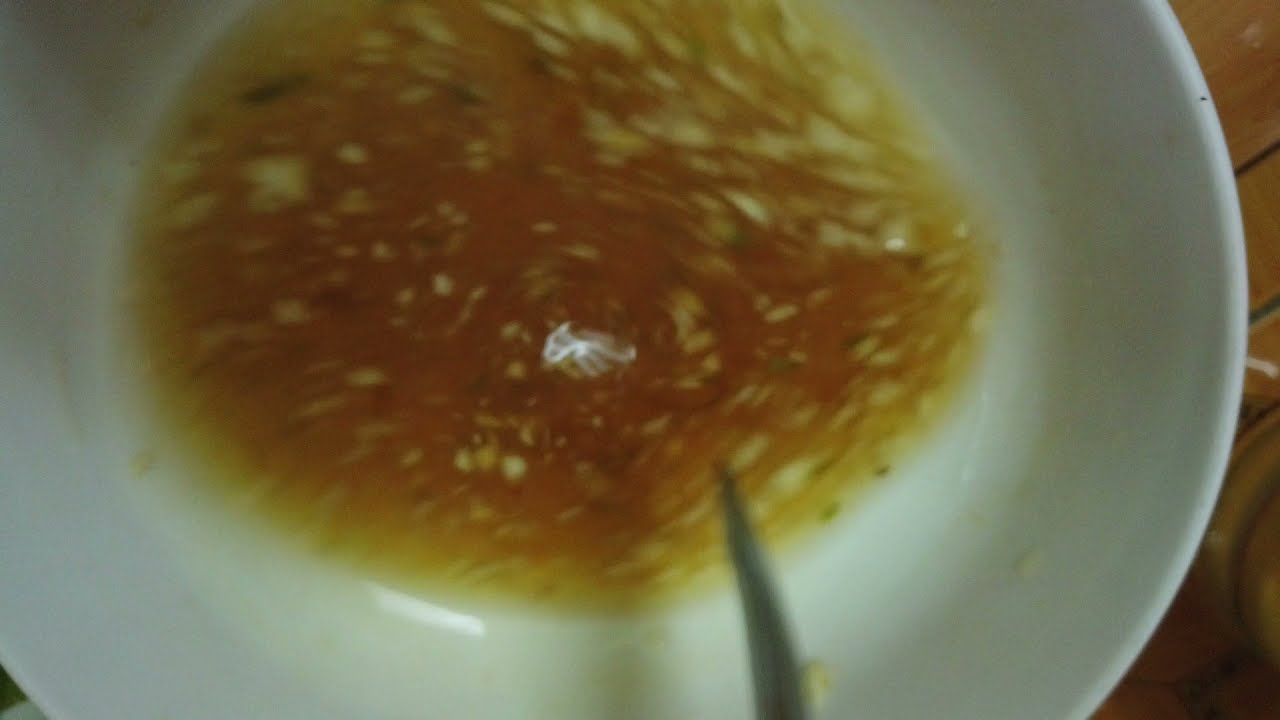The image showcases a white bowl, centrally positioned on what seems to be a brown wooden table with visible black lines separating the wood planks. The bowl contains an orange liquid, likely a soup, with small, distinct pieces of white and green scattered throughout. Some of the liquid has been consumed, revealing a reflective patch towards the bowl's center. A silver spoon, barely discernible due to motion blur, is inserted into the bowl on the center-right side. The image, taken from above, captures not only the culinary contents but also hints of light reflecting off the soup's surface. The scene is set indoors, offering a snapshot of a partially finished meal.